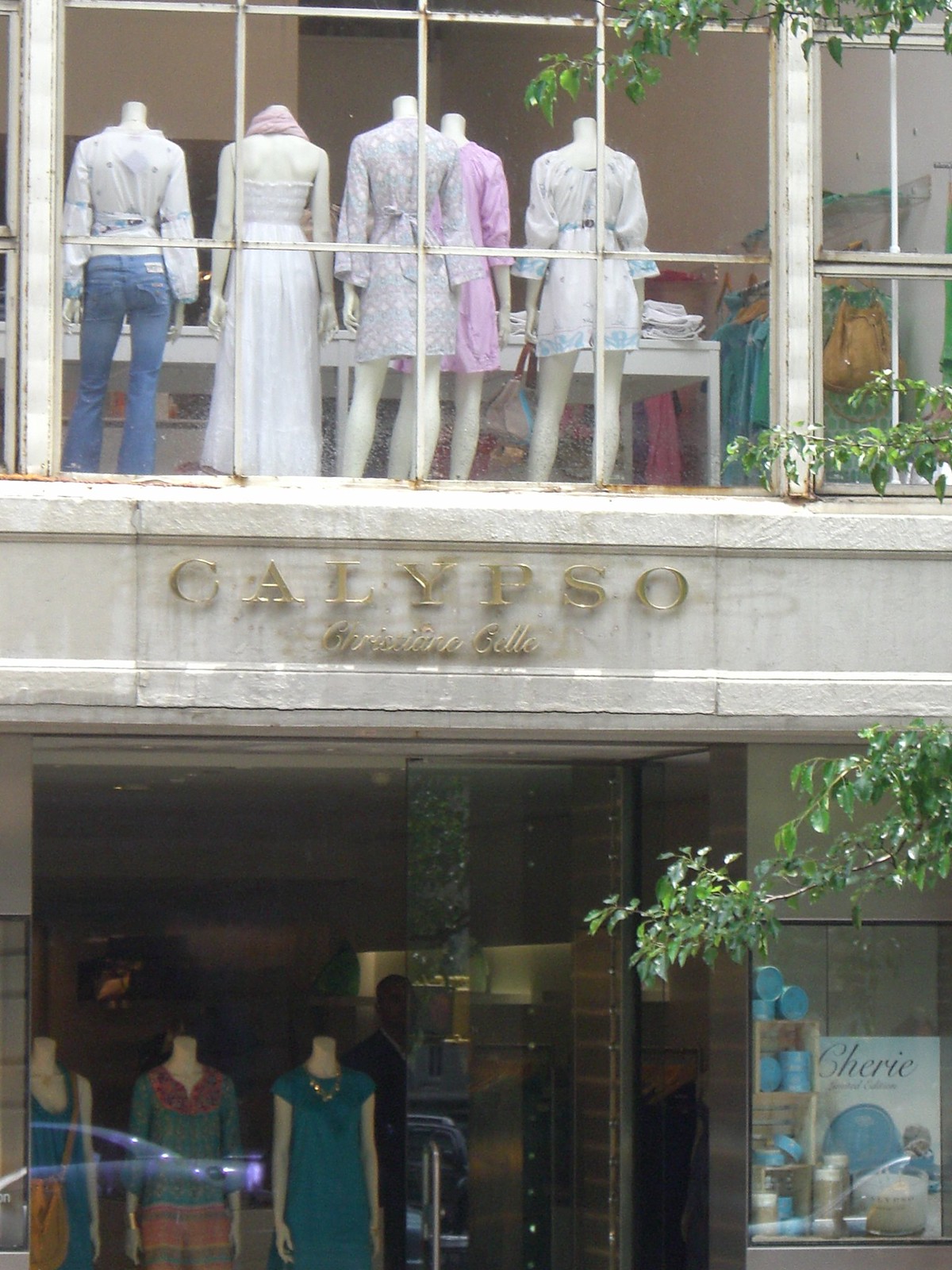The image captures the two-story exterior of a clothing shop named "Calypso," prominently displayed in gold lettering above the glass entrance, with additional cursive gold text underneath. It's midday, and the photograph showcases both the ground and first floors through large window displays. On the ground floor, a glass door is flanked by two windows. Through these windows, three headless mannequins are visible, all dressed in blue outfits; one mannequin is adorned with a purse slung over its shoulder. To the right, a display case contains several blue containers. 

The upper floor features five more headless mannequins facing away, clothed in various outfits; noteworthy is one mannequin dressed in blue jeans and a white long-sleeve top. Additionally, behind the mannequins are a visible clothing rack mounted on the wall and a table abundantly covered with more clothing. The store is surrounded by an urban environment, hinting at a bustling city setting. The wide array of colors including white, gray, brown, blue, pink, green, teal, orange, red, and purple, adds vibrancy to the scene. A hint of other cityscape elements frames the shop.